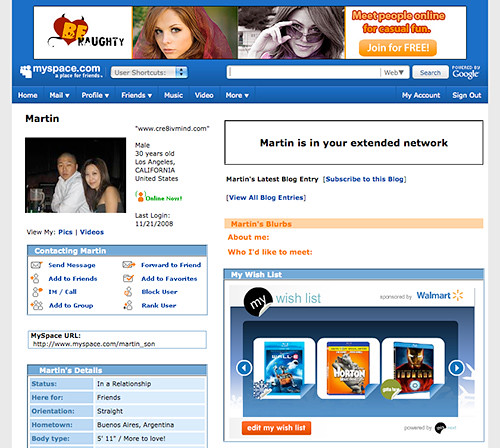Here is a cleaned-up and detailed caption for the described MySpace screenshot:

---

Screenshot of a vintage MySpace page, featuring a MySpace.com graphic prominently displayed at the top. At the very top of the page, a vibrant advertisement with the text "Be Naughty" is highlighted, showcasing a heart with devil horns and a tail. Accompanying this ad, there is an image of a red-haired woman and a black-and-white photo of another woman peering over her sunglasses. The ad encourages users to "meet people online for casual fun" and offers a free signup through an orange button.

Below the ad, navigation options are visible, including "Home," a semi-visible option due to poor resolution, "Profile," "Friends," "Music," "Videos," and more. A search bar powered by Google is also present, currently empty. A user drop-down menu offers shortcuts among other options.

The main focus of the page is a MySpace profile for a user named Martin, with a link to www.creativemind.com. Martin is identified as a 30-year-old male from Los Angeles, California, USA, with his last login dated November 21, 2008. The page provides various interaction options such as sending a message, adding to friends, instant messaging, calling, adding to a group, forwarding to a friend, adding to favorites, blocking the user, and ranking the user. A grainy photograph depicting an Asian-looking man in a white shirt sitting next to a dark-haired woman (possibly Caucasian) accompanies his profile.

Further details about Martin include his status ("In a relationship"), intention ("Here for friends"), orientation ("Straight"), hometown ("Buenos Aires, Argentina"), body type ("5'11" More to love"). A bold message on the right-hand side declares, "Martin is in your extended network," with options to view, subscribe to, or learn more about his blog.

At the bottom right corner, there's an advertisement for Walmart featuring video games or movies. Titles include "Iron Man," "Horton Hears a Who," and an unidentified third item.

---